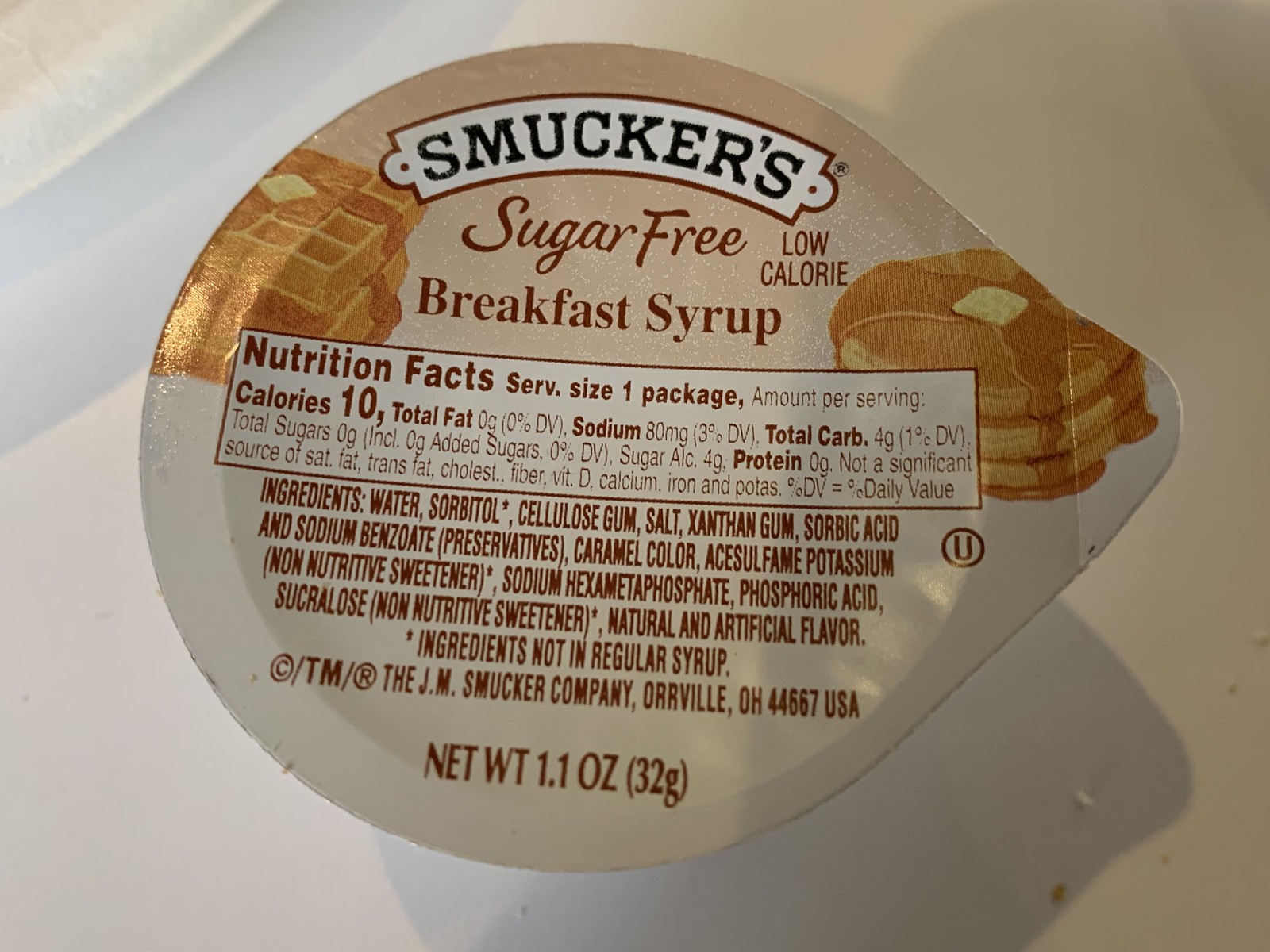This image is a detailed top-down view of a small packet of Smucker's Sugar-Free Breakfast Syrup, commonly found in diners or restaurants. The packet features a circular label with a pointy end on the right, serving as a pivot point. Across the top of the label, it reads "Smucker's Sugar-Free Breakfast Syrup," emphasizing its sugar-free, low-calorie nature. On the left side of the label, there's an image of stacked waffles topped with a slice of butter and syrup flowing down the middle. On the right side, there’s a depiction of pancakes, also topped with butter and drizzled with syrup.

Central to the label, enclosed in a rectangular area, are the nutrition facts: 10 calories, 0 grams of total fat, 80 milligrams of sodium, 4 grams of total carbohydrates, 0 grams of total sugars and added sugars, 4 grams of sugar alcohol, and 0 grams of protein. It notes that it is not a significant source of fat, trans fat, cholesterol, fiber, vitamin D, calcium, iron, and potassium. 

Below the nutrition facts, the list of ingredients is displayed in brown print, detailing components such as water, sorbitol, cellulose gum, and various preservatives and sweeteners. The packet also mentions the copyright and trademark of The J.M. Smucker Company, based in Orrville, Ohio, and shows a "U" within a circle, indicating kosher certification. The net weight is listed at the bottom as 1.1 ounces or 32 grams. The packet itself casts a shadow in the bottom right-hand corner and sits on a white surface.